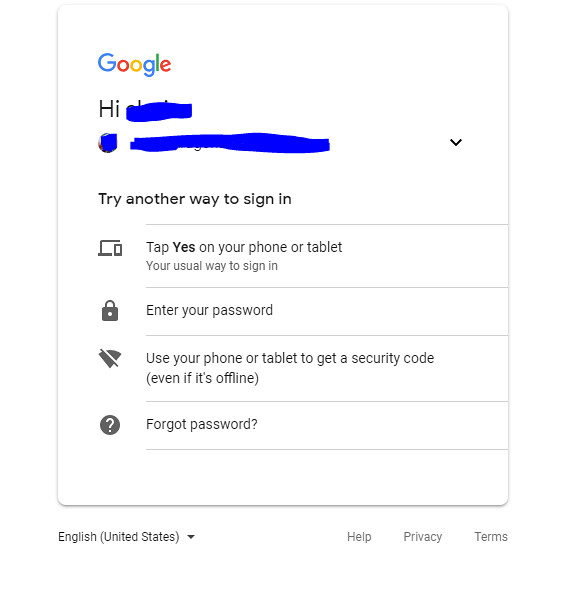This screenshot captures the sign-in screen of a Google account on a smartphone. At the top, the familiar Google logo is prominently displayed, followed by a greeting, "Hi." The name of the person trying to sign in has been redacted using a blue marker. Directly below, the screen prompts the user to "Try another way to sign in." This message is followed by a security prompt that offers several sign-in methods: tapping "Yes" on a smartphone or tablet, entering a password, or using a phone or tablet to get a security code. An option to recover a forgotten password is also available. Icons representing a smartphone and a lock are displayed below the text, reinforcing the security-focused nature of this sign-in process. The overall design is clean and standardized, typical of Google's user interface for account security alerts.